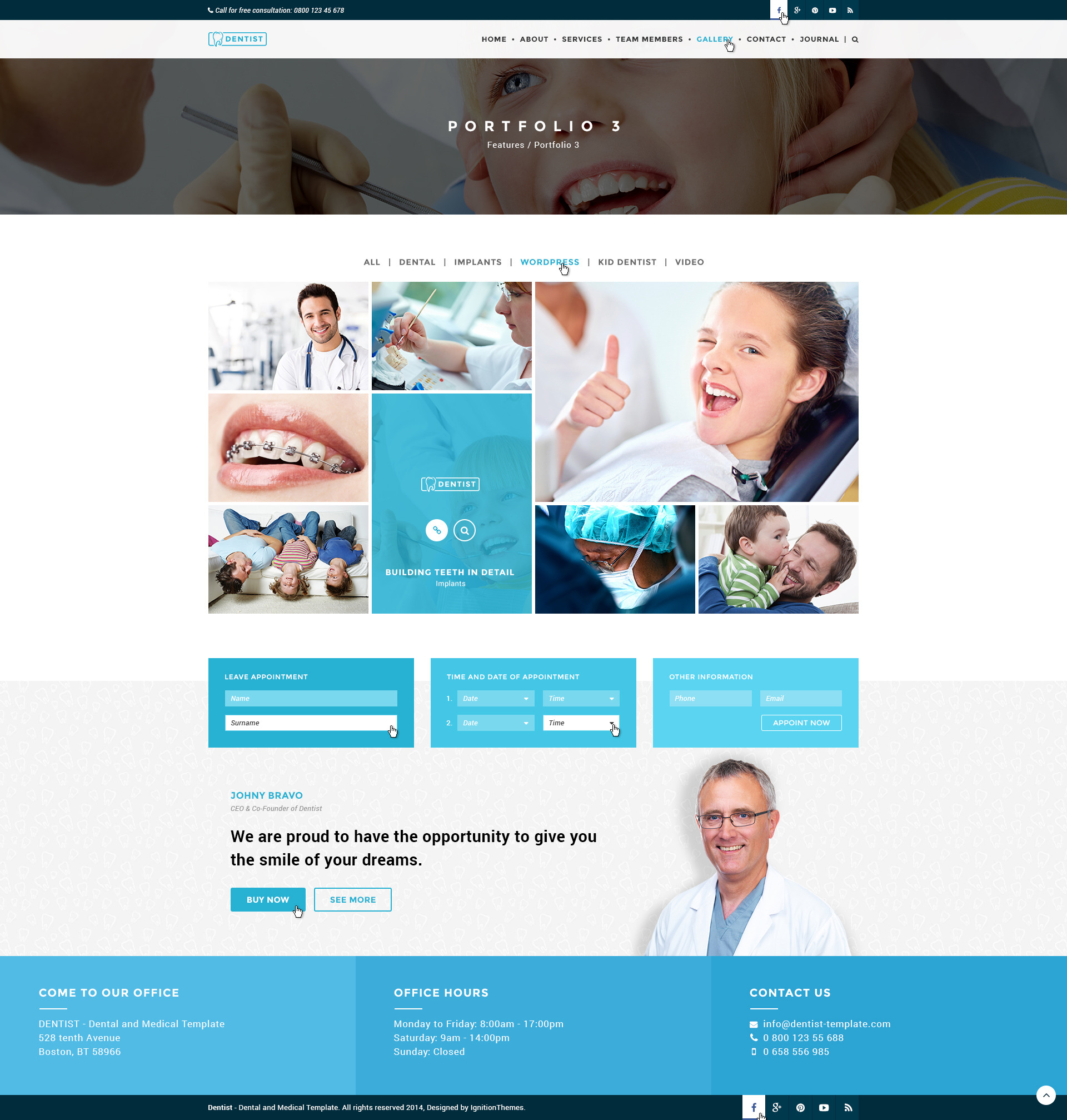This is a vertical rectangular photograph of a webpage. At the top of the image, there is a small horizontal white rectangle featuring a navigation menu in all black capital letters. The menu items listed are 'Home,' 'About,' 'Services,' 'Plan Members,' and an unreadable item in turquoise. Following that are 'Contact' and 'Journal.'

Beneath the menu, there is a horizontal rectangular image displaying the word 'PORTFOLIO' in white, all-capital letters, overlaying the number three and some small text beneath it. The image, slightly grayed out, depicts a woman with her mouth open, possibly undergoing a dental procedure. Hands are positioned on either side of her face, and a dental instrument and a bit of the practitioner's chin are visible in the upper left corner.

Below this, another horizontal rectangular image contains multiple smaller images in both horizontal and vertical orientations. These include a doctor with a stethoscope, a close-up of a person's mouth with braces, and a girl sitting in a chair wearing a dental bib and giving a thumbs up, among other similar visuals.

Further down, there are three small turquoise rectangular images with text that is too small to read clearly. Beneath these, a bold black font states, "We are proud to have the opportunity to give you the smile of your dreams." Following this, there are two horizontal rectangular buttons: a bold white-lettered 'BUY NOW' button, and a 'SEE MORE' button with turquoise lettering on a white background. To the right of these buttons, there is a man dressed in a white doctor's coat and glasses.

At the bottom of the webpage, a section with a solid turquoise background displays the phrase "COME TO OUR OFFICE" in white, all-capital letters. Underneath, in smaller lowercase letters, is the office address, although it is too small to discern. The final sections are titled 'Office Hours' and 'Contact Us.'